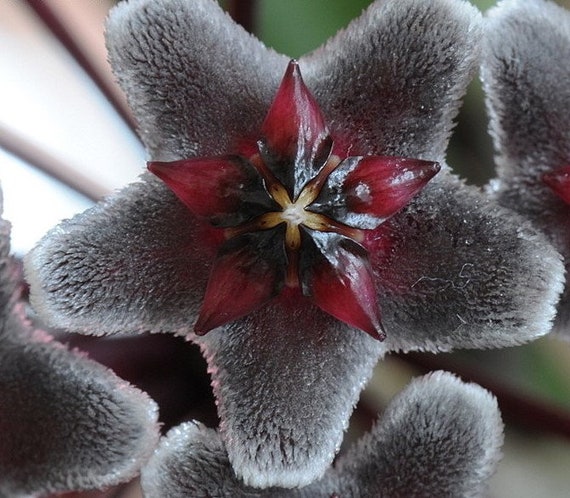The image is a detailed, close-up photograph of a captivating flower, composed of multiple layered shapes resembling stars. The outermost flower is fuzzy and gradient-toned from a light white to dark gray, evoking the softness of fur. Nested within its star-like form is a bright red flower, mirroring the star pattern but smaller, with its points interlocking with the larger flower's gaps. At the very center of this red star-shaped flower lies a yellow bulb, serving as the apparent center and nectar source for both floral structures. The square-shaped image focuses closely on the intricate layers of this plant, with the background blurred out, allowing the geometric beauty and vivid colors of the flowers to dominate the view. Edges of surrounding similar plants are faintly visible around the sides, adding a sense of repetition and depth to the composition.